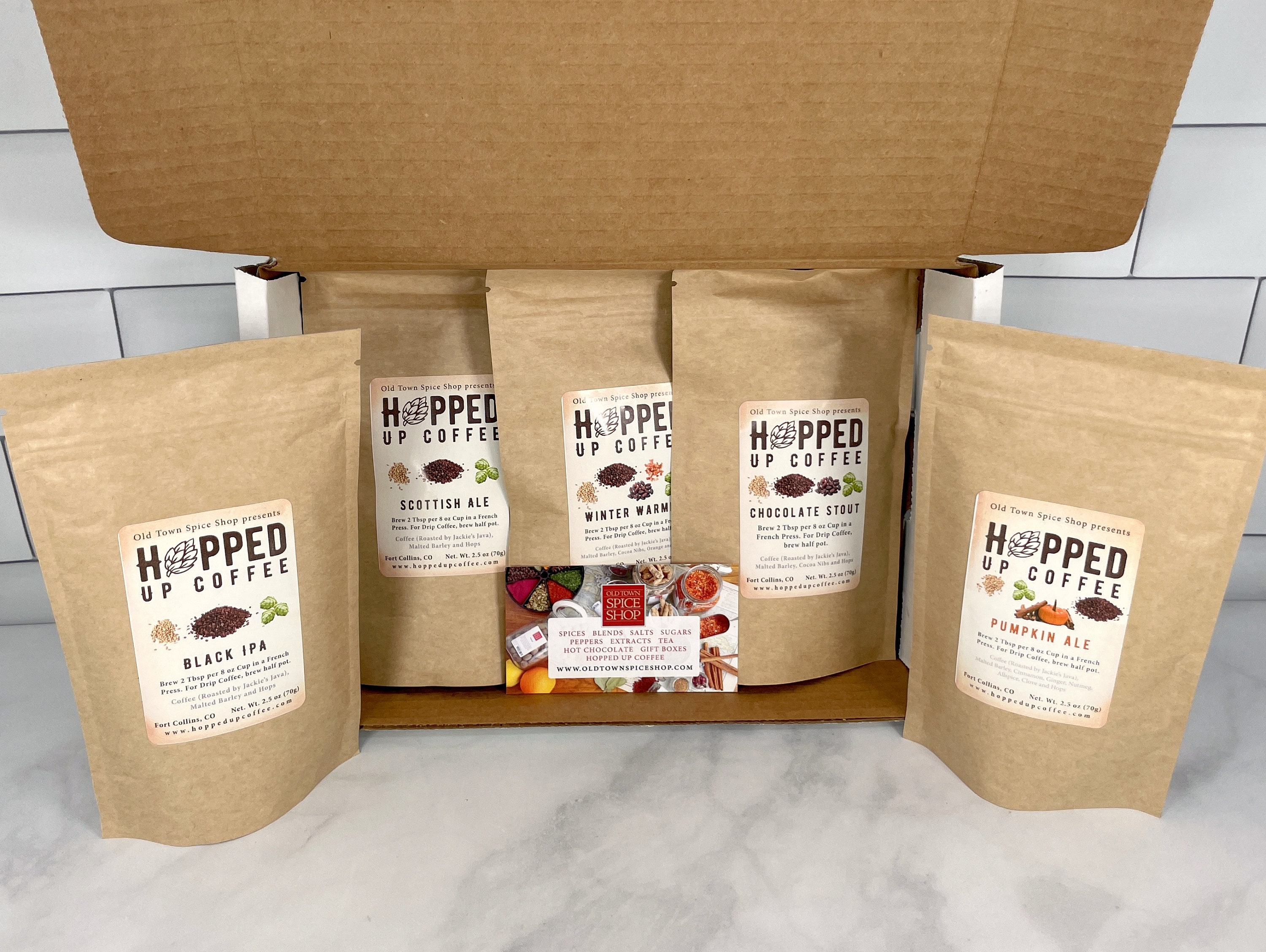Displayed on a white and gray granite countertop with a white backsplash, this photograph features a sample box of Hopped Up Coffee, a small business specializing in unique coffee blends. The sample box contains five biodegradable light brown pouches, each labeled "Hopped Up Coffee" with a distinctive logo where the 'O' is replaced by a pine cone. Underneath the brown text label, the pouches feature images of different colored beans and flavors, including Black IPA, Scottish Ale, Winter Warm, Chocolate Stout, and Pumpkin Ale. In the center of the composition, three of the five pouches are neatly arranged inside a white cardboard box. Accompanying the coffee pouches is a card from Old Town Spice Shop, adorned with a red border and white text, providing an additional touch of artisanal appeal and possibly offering purchasing information. The setup suggests this could be a promotional photograph for a gift box or an introductory kit available on the company's website.